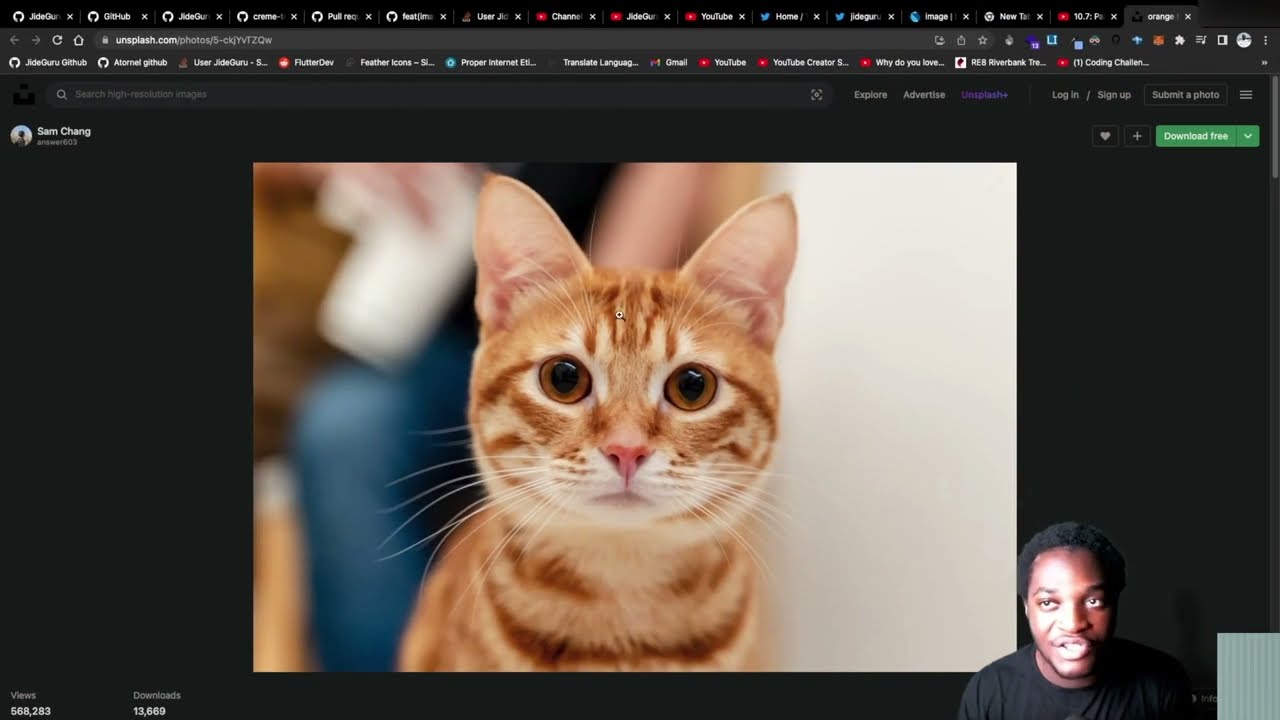In the image, prominently displayed at the center, is an orange tabby cat with darker brown stripes, white accents around its eyes and mouth, and pointed ears. The cat, which has brown eyes and white whiskers, is staring directly at the camera. Behind the cat, there is a slightly out-of-focus person wearing a black t-shirt and blue jeans, seated on a brown wooden bench and holding a white cup. To the right of the cat, a white wall is visible. This scene is displayed on a black computer monitor.

Overlaying the lower right corner of this cat image is the face of a dark-skinned man with black curly hair, also wearing a black t-shirt, appearing as if he is talking. This setup resembles a screen capture of a web page, complete with navigation bars at the top in white text on a black background. Notably, in the top left corner of the screen, it states that "Sam Chang" is the poster of the picture. The man on the screen might be discussing a topic, potentially related to pet adoption, given the context of the image. Additionally, multiple open tabs are visible on his computer screen.